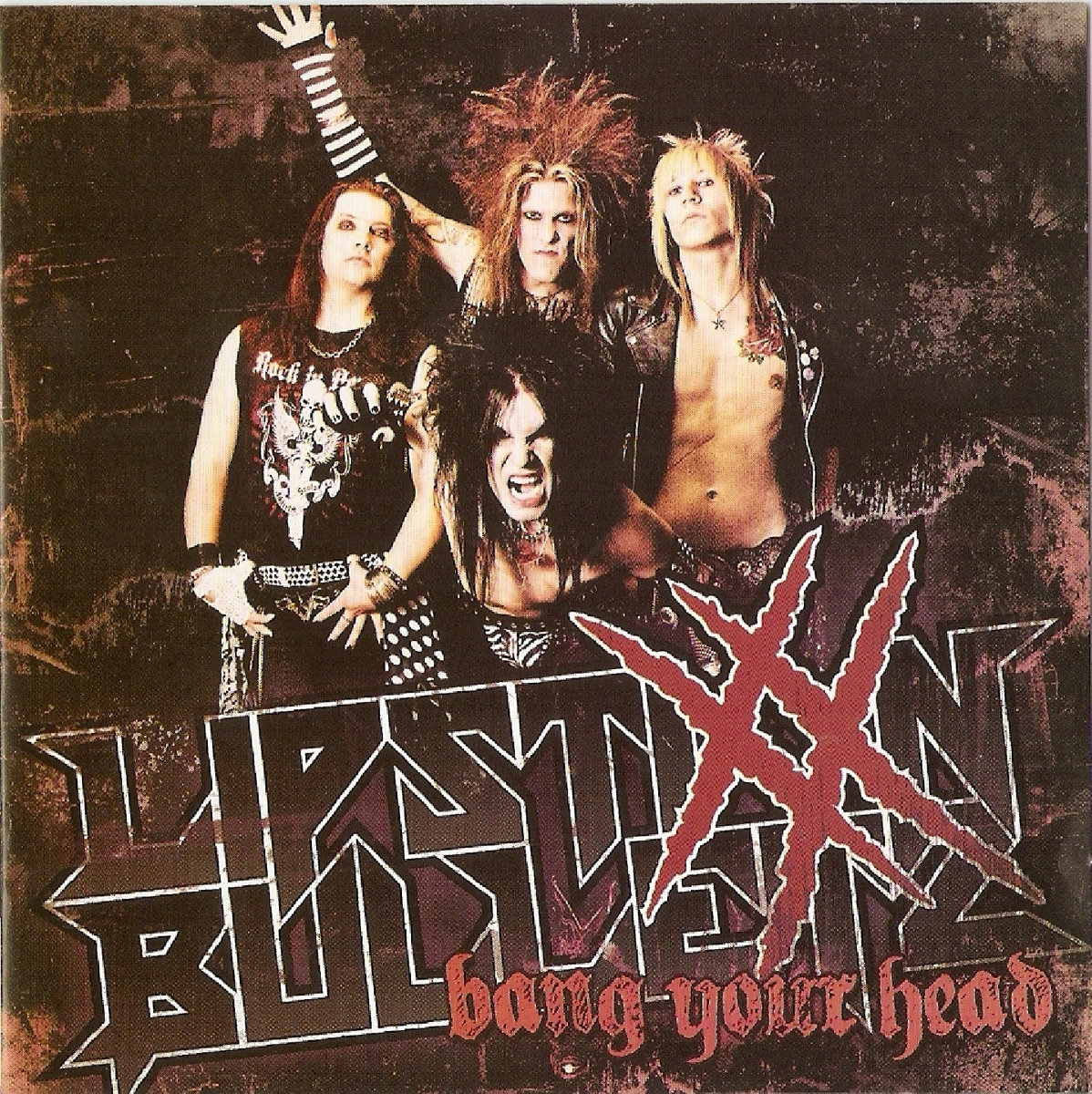This detailed album cover features a heavy metal band called "Lipsticks and Bullets," with "Lipsticks" ending in two stylized red Xs and "Bullets" ending with a Z. The album title "Bang Your Head" is prominently written in a gothic, stylized red font at the bottom right. The artwork has a faded, pen-and-ink illustration style with fuzzy shading and a dark brown and red background, evoking an old, gritty feel, reminiscent of dried blood.

The cover showcases the four band members, all facing the camera with intense expressions. The frontman, standing prominently and screaming at the viewer, sports long black hair and white face makeup, giving him a ghastly, pale appearance. His ensemble includes zebra-printed underwear over leather pants, accentuating his dramatic look.

To his side, another member with long blonde hair wears an open leather jacket and low-cut pants, revealing his bare chest. Behind them, a band member with spiky red hair wears black and white striped fingerless gloves that extend from his elbows to his palms, adding to the eclectic visual. Partially obscured, he has a scowl directed at the camera. 

The fourth member, appearing on the left, has a sleeveless shirt emblazoned with a skull and a winged dagger, accessorized with a jeweled belt and long pants. His thumbs are tucked into his belt loops, and he sports a rock 'n' roll attitude, complete with black nail polish.

The overall effect of the cover suggests a raw and rebellious energy, typical of the heavy metal genre, enhanced by the band’s spiky hairdos, leather and metal attire, and their fierce, snarling expressions.